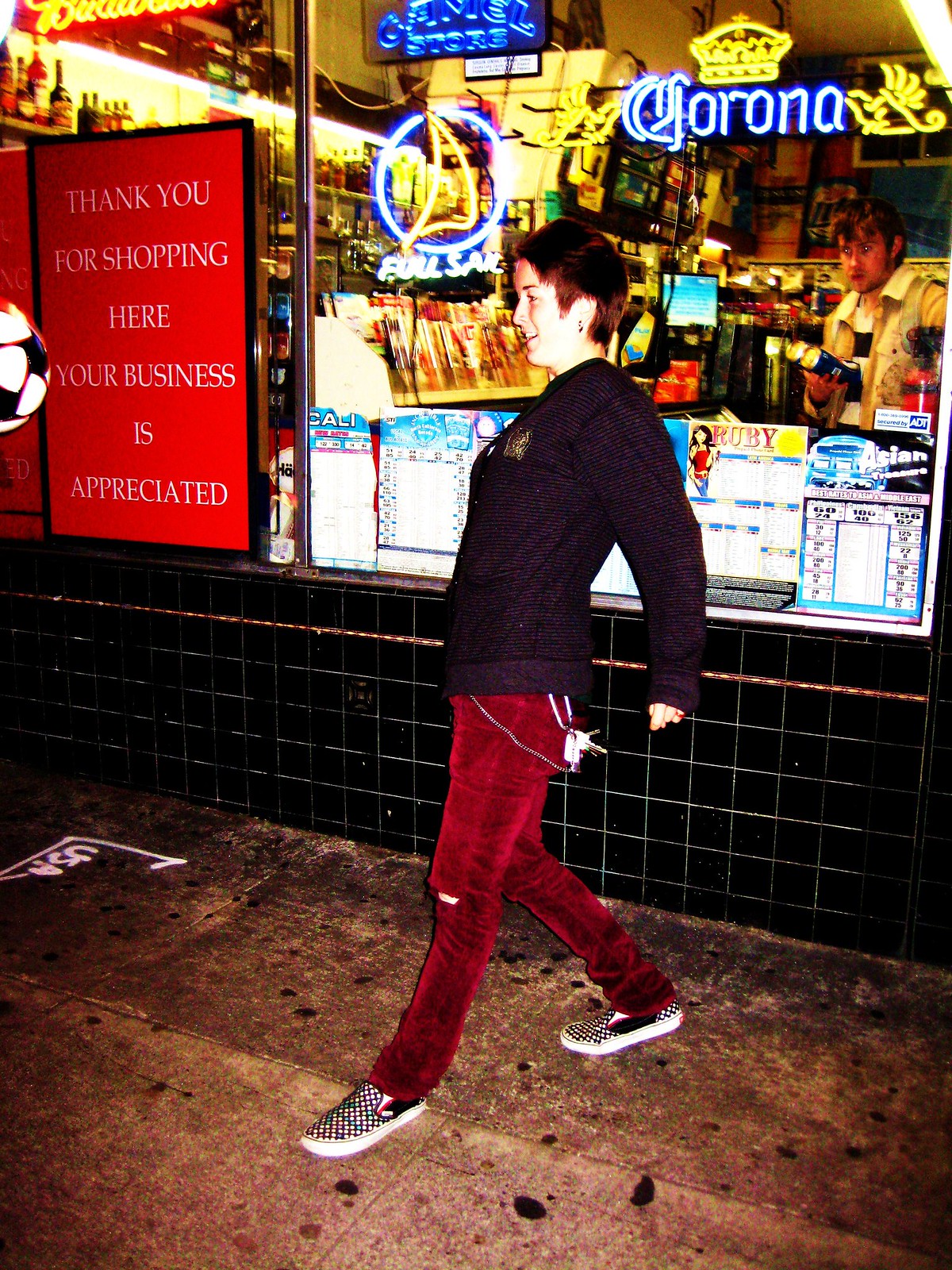In the photograph, a young woman stands in front of a liquor store. She has short, reddish-brown hair styled almost like a man's cut and a light skin tone. The woman is dressed in long, red corduroy pants and a dark, long-sleeved top. She wears checkered skate shoes with white rims, with her left leg extended forward and her right leg positioned behind her, giving her a slightly leaning back posture. Her left arm rests just slightly behind her.

The storefront features small black square tiles at the bottom and an orangey, mottled pavement in front. A distinctive sign to the left of the image reads, "Thank you for shopping here. Your business is appreciated," displayed in white letters on a red background bordered with black. Neon signs, including one for Corona, are visible in the window. Inside the store, a person can be seen looking out towards the woman. A tile and sidewalk connection completes the foreground, merging into the pavement. The woman's casual yet distinct appearance, coupled with the details of the storefront and signage, creates a vividly urban scene.